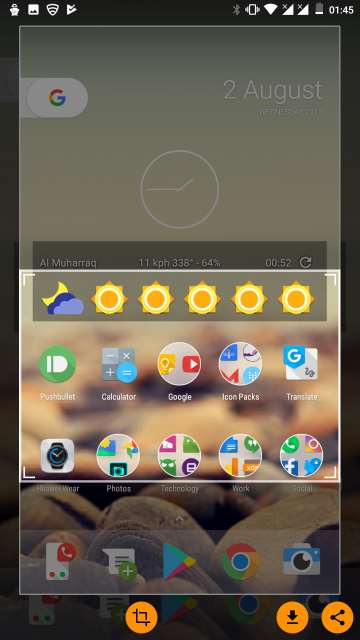The image depicts a screenshot currently being edited on a mobile device, evident from the standard icons at the top indicating Bluetooth connection, time, Wi-Fi signal, network connection, and battery life. The screenshot showcases a user's phone homepage, complete with the date, time, various app icons, and widgets for weather, a clock face, and shortcuts to essential tools like the internet and camera. A semi-transparent rectangular box obscures part of the image, signifying an area being selected for cropping. Within this selection, a square section remains visible, concentrating on the circular icons representing different apps and folders, suggesting that this portion is intended to be retained from the original screenshot.